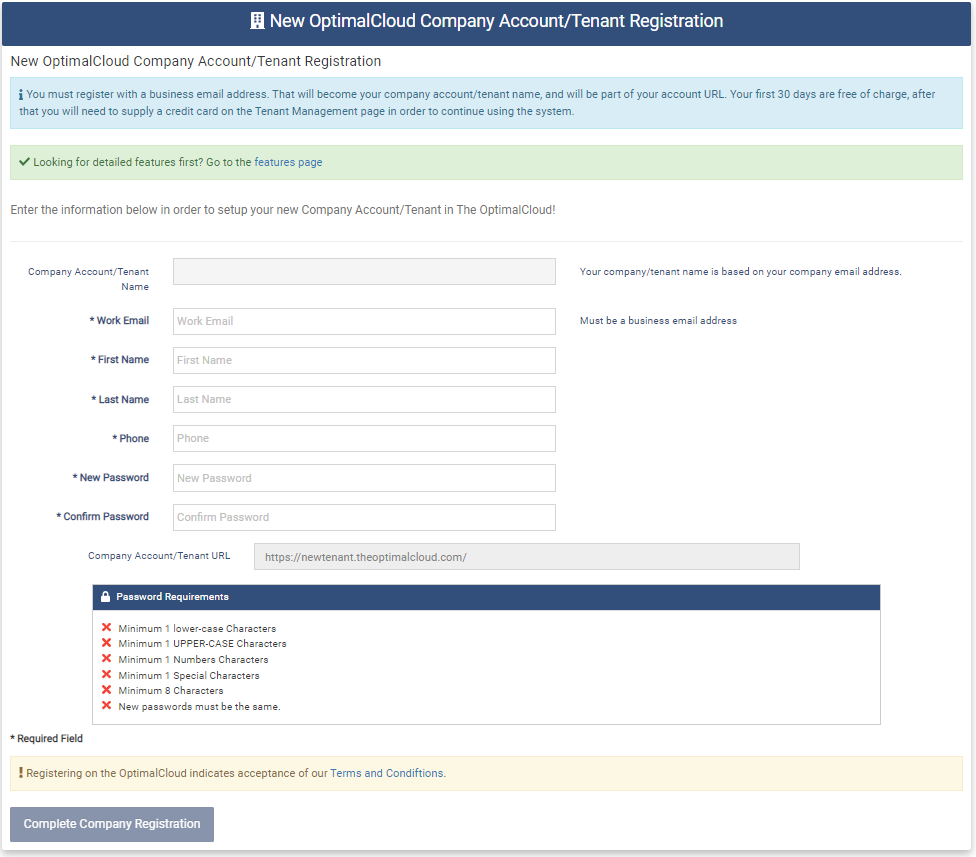The image depicts a web page designed for setting up a new company account. The layout features a clean, white background with a blue border at the top. The top blue bar prominently displays the text "New Optimal Cloud Company Account for its Last Tenant Registration" in white letters, which is repeated just below in blue text. A blue information box explains the requirement to register a business email address, followed by a green information box advising users to visit the features page, highlighted with a blue hyperlink for detailed features. 

Below these boxes, instructions guide users to enter their information to set up a new account. The form fields include "Company Account Name," "Work Email," "First Name," "Last Name," "Phone Number," "New Password," and "Confirm Password." Additionally, password requirements are listed to ensure users create a secure password. Finally, a dark grey button labeled "Complete Company Registration" in white letters is situated at the bottom left of the page, ready for users to submit their information.